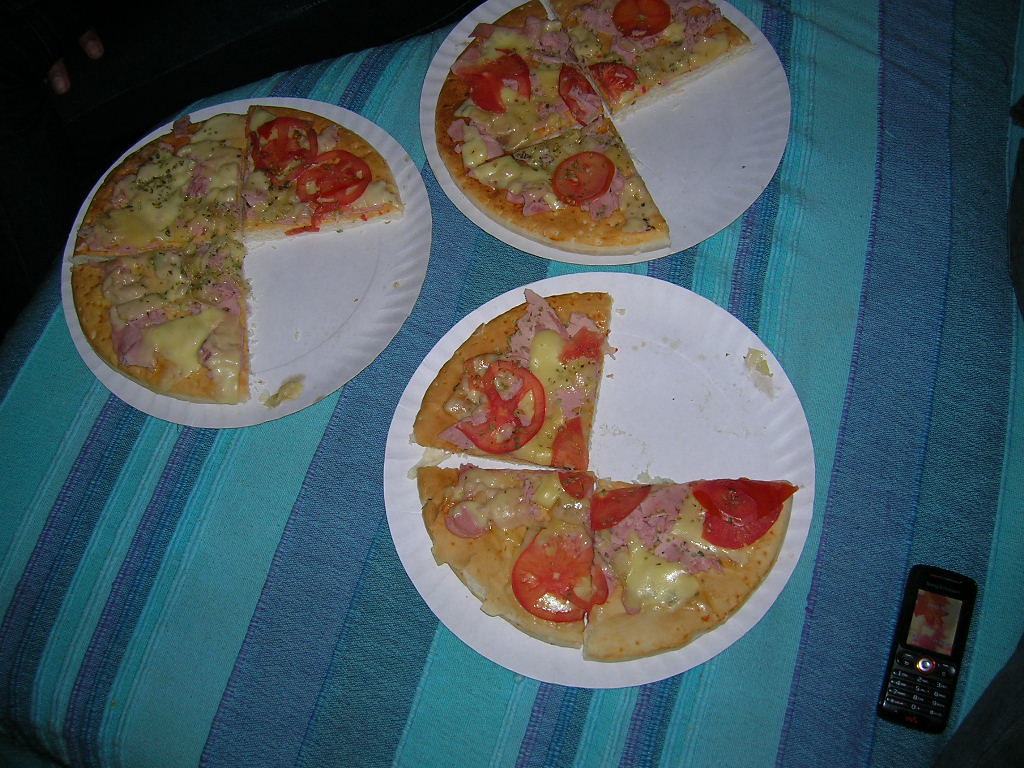The image depicts an indoor, dimly lit scene, possibly taken in the evening, showing three white paper plates with pizza, each placed on a striped blue and teal cloth backdrop, which could be a tablecloth, blanket, or padded cushion with a unique shape. Each plate holds three triangular slices of thin-crust pizza, one slice already missing. The pizza flavors appear to vary slightly: most slices are topped with cheese, Canadian bacon, and tomato, while two slices lack tomato and instead have extra cheese. Amongst the plates in the bottom right corner lies an old-style black Nokia cell phone with a small screen, typical of models from the mid-2000s to 2010, adding a nostalgic touch to the scene. The overall appearance of the image is somewhat muted and dated, suggesting it might have been taken some time ago.